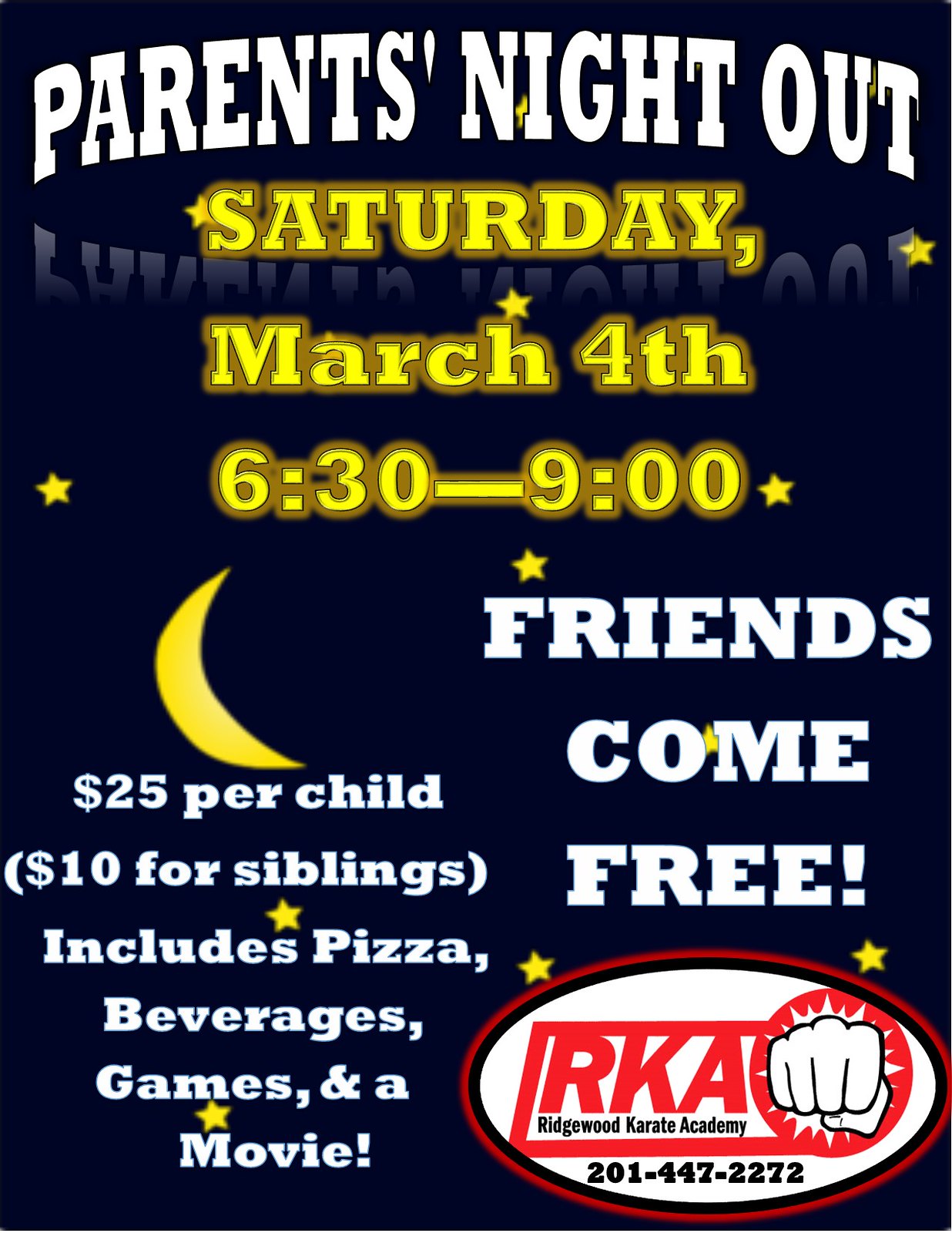The poster for the event titled "Parents Night Out" is a vertical rectangular image with a black background featuring scattered gold stars and a gold crescent moon. At the very top, in white text, it announces "Parents Night Out." Below, in yellow letters, it details "Saturday, March 4th, 6:30 to 9:00 PM." Positioned to the right, in large white letters, it states "Friends Come Free." On the lower left corner, under the crescent moon, it mentions the pricing details: "$25 per child, $10 for siblings." This section also includes the benefits of attending the event: "includes pizza, beverages, games, and a movie." The bottom right corner of the poster features the logo and contact information for the event sponsor, Ridgewood Karate Academy (RKA). The logo is a red-bordered oval with a white interior, showcasing a white-outlined drawing of a fist moving forward within a red circle. Beneath the logo, it reads "RKA, Ridgewood Karate Academy," followed by the phone number "201-447-2272."